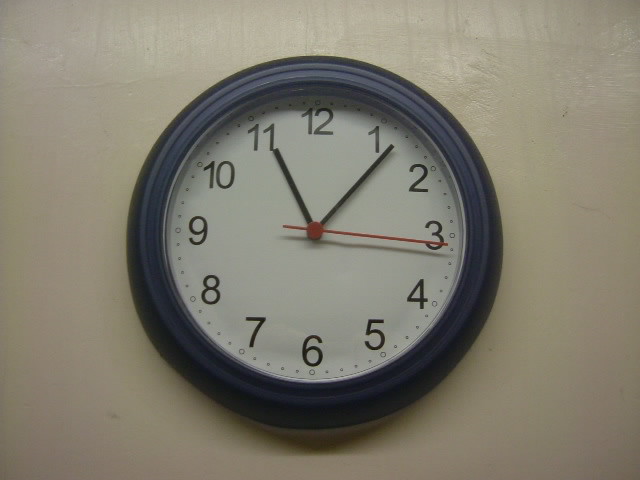This photograph captures a navy-colored round clock mounted on an off-white wall. The face of the clock features a crisp white background with black numbers and two black hands, alongside a red second hand. Small black circles adorn the perimeter of the clock face. Visible beneath the clock is a projected shadow against the wall, with additional shadowing near the top, around the number 12. The wall above the clock is marred by what appear to be moisture streaks, and there is a noticeable patch of dirt on one side of the image, further emphasizing the aged and slightly neglected appearance of the setting.